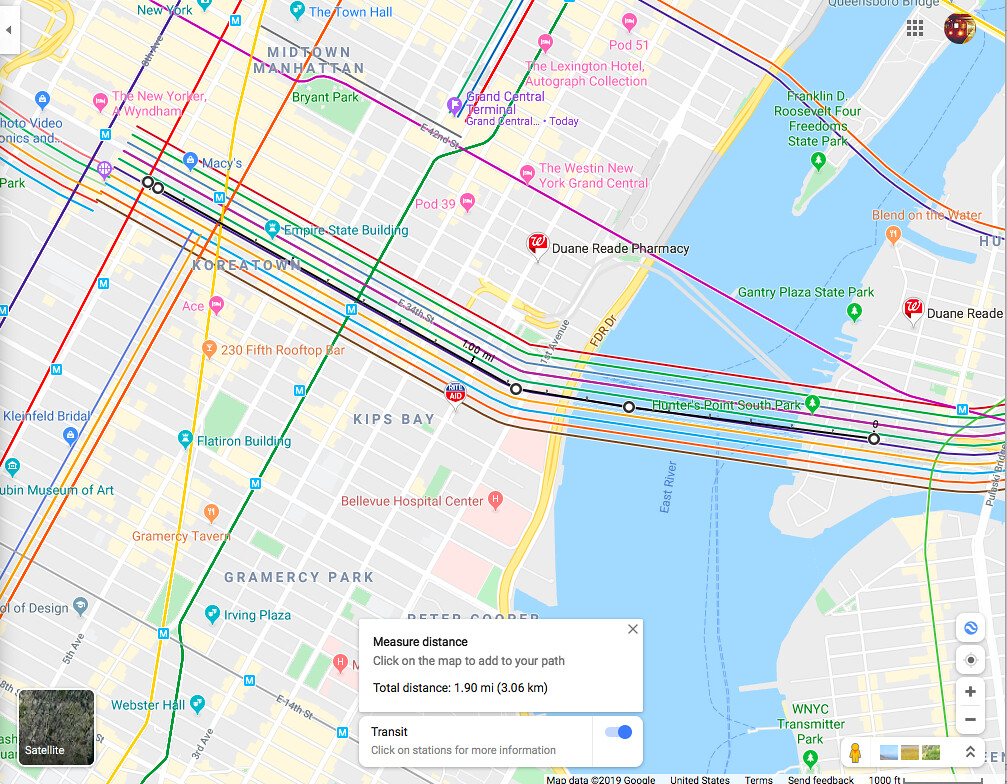**Detailed Caption:**

This image depicts a detailed and colorful map of New York City, specifically highlighting Midtown Manhattan. The map is crisscrossed with numerous roads and paths, and includes a measuring tool that allows users to click on the map to add points to their path, with a total displayed distance of 1.9 miles. Key features indicated on the map include WNYC Transmitter Park, Kips Bay, and Bellevue Hospital, confirming its focus on New York City.

Notable landmarks such as the Empire State Building and Macy's are prominently marked, providing essential information for navigating the city. Additional points of interest, like Duane Reade pharmacy, add practical value for those seeking specific services. The map also prominently features transit information, showing various stations and inviting users to click on them for more details.

The map is vibrant, with text and labels in pink, orange, red, and green, making the different elements easily distinguishable. Midtown Manhattan is clearly labeled, aiding in orientation. There is also an option to switch to a satellite image for a more detailed and realistic view of the area. The map effectively balances informational content and visual appeal, offering a comprehensive overview of Midtown Manhattan and surrounding areas.